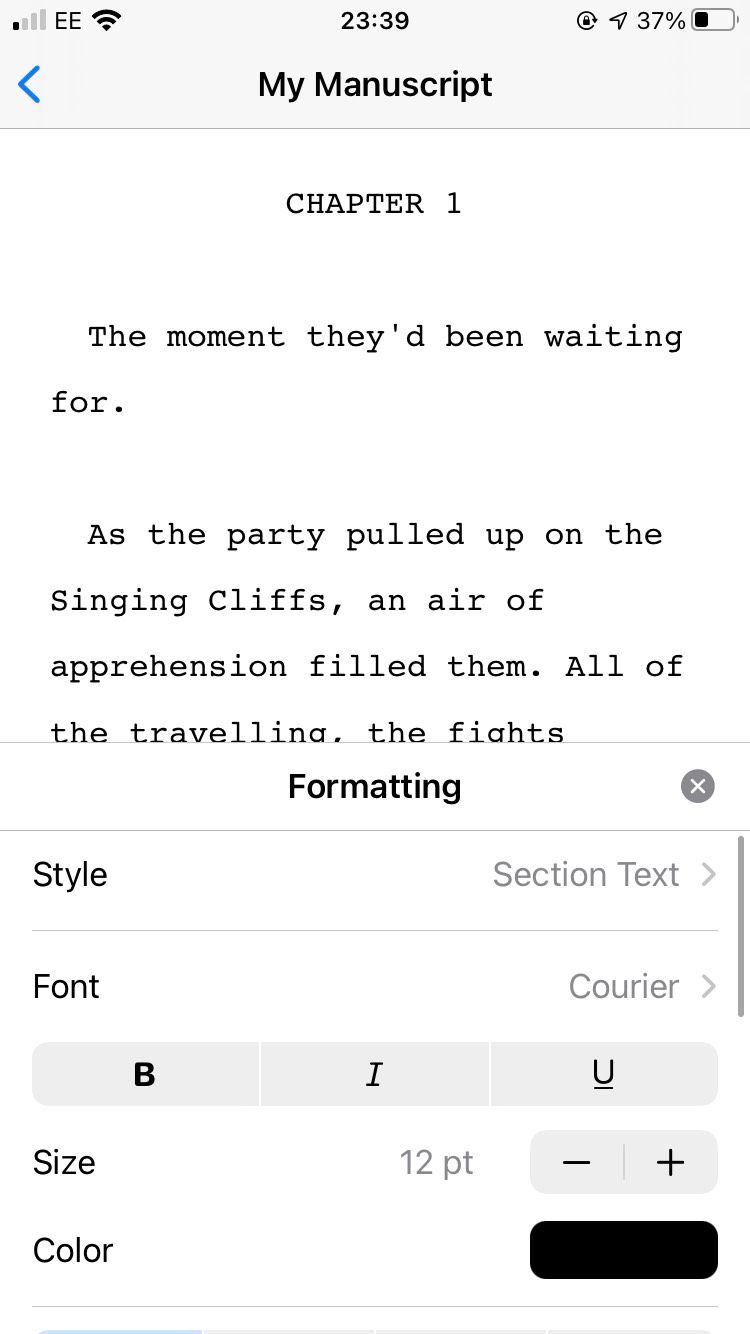This is a detailed screenshot of a phone application. At the very top of the screen, the time is displayed as 23:39 and the battery is at 30% power. The main part of the screen shows the beginning of a manuscript labeled as "Chapter One" with the title "The Moment They've Been Waiting For". The text describes a party arriving at the singing cliffs with a feeling of apprehension building among them. Due to the constraints of the screen, the text cuts off after mentioning their extensive travels.

Below the manuscript text, a section labeled "Formatting" is visible, with an 'X' icon on the right-hand side for closing the section. This area contains options laid out in horizontal rows. The first row offers formatting options such as style selection, text settings, and forward navigation buttons. The subsequent row features buttons for bold, italicize, and underline functions.

Further down, there's an option to adjust text size, which is currently set to 12 points, with buttons to increase or decrease the size. Following that, there is a color selection box indicating that black is the selected text color. At the bottom of the screen, multiple gray bars are present, with the first quarter highlighted in light blue, indicating that the user is on the first of several formatting screens.